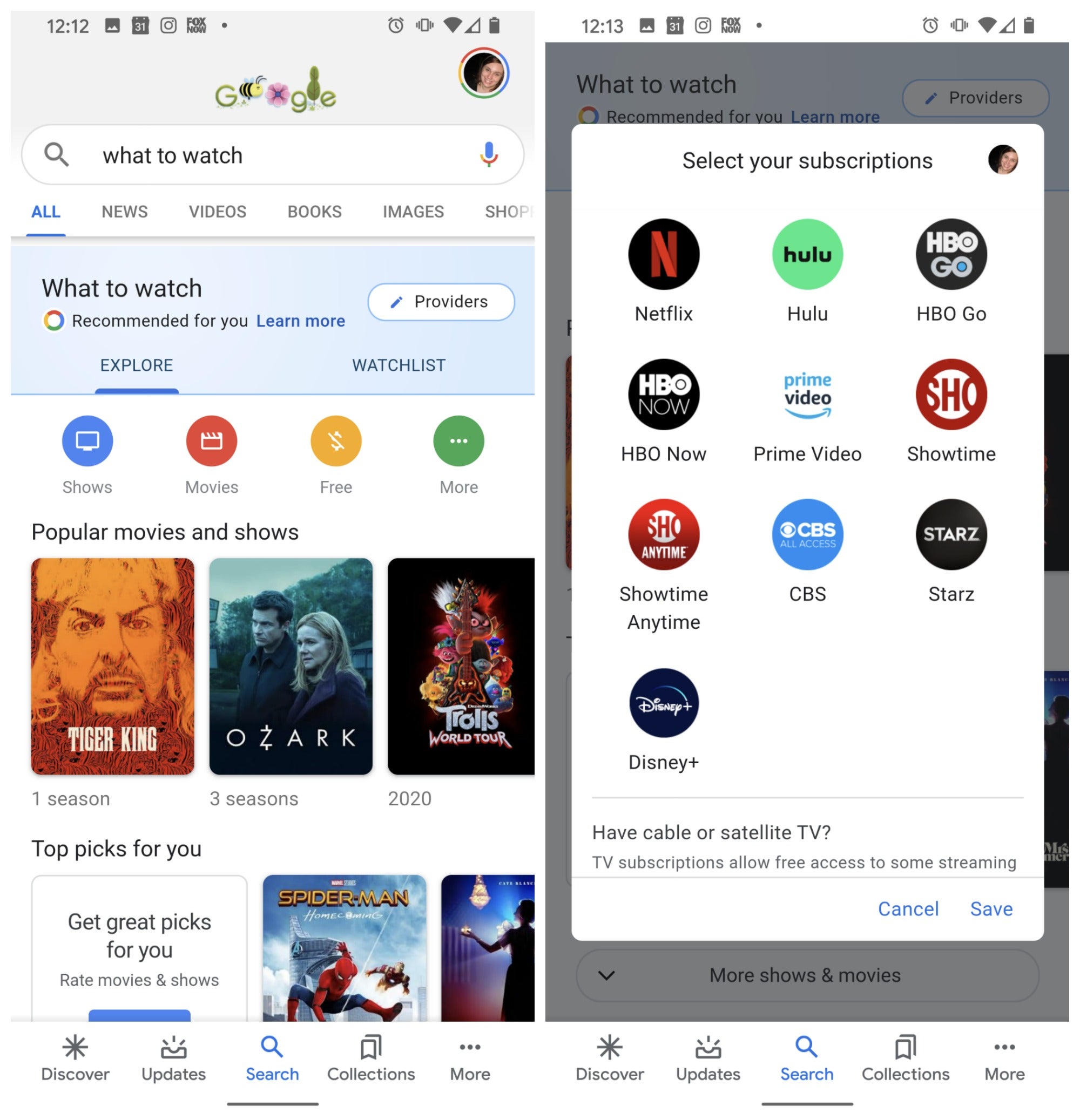The image features two vertically aligned smartphone screenshots placed side by side. The left screenshot displays a Google search page. At the top, the header shows the time as 12:12 PM, along with various status icons including timer, alarm, vibration, Wi-Fi, signal strength, and battery level. The user profile icon is visible in the top right corner. The word "Google" is whimsically styled, with a "B" replacing one of the "O"s and a small tree or flower substituting the "L". Below this, the search bar contains the query "what to watch". The search results include a variety of movie thumbnails and recommendations.

The right screenshot appears similar but with a notable difference: the page has been grayed out and an overlay is present. This overlay features a header titled "Select Your Subscriptions" and outlines a list of 10 streaming service providers, each represented by their respective names and icons, for the user to choose from.